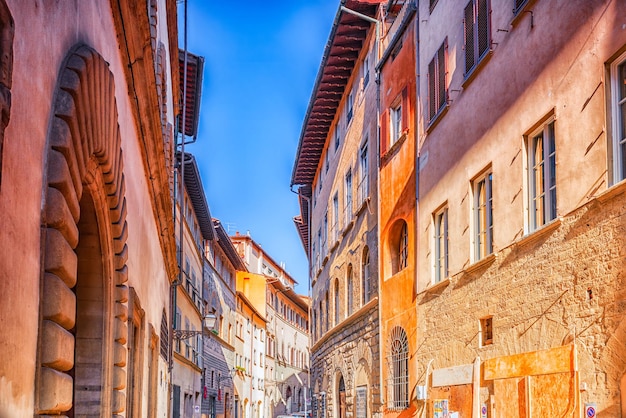The image presents a detailed view of the upper sections of a narrow street flanked by buildings, illuminated by bright sunlight under a clear, vibrant blue sky. On the right side, a taller building with at least three visible floors displays light brown walls on the bottom floor, decorated with a single small window, and morphs into tan and light brown hues ascending to a purple-tinted upper section. The second and third floors are lined with four windows each. Notably, there is a middle section with striking orange walls, featuring two arch-shaped windows on the lower levels and a rectangular window above.

On the left side, the forefront building is slightly shorter with a distinguished two-story high archway that features decorative brown tiles around its edges. This building also has two windows on the front facade. Behind it, buildings continue in a pattern consistent with light-colored or white walls, with second and third floors peppered with various windows. Both sides exhibit shadows cast by the sun, enriching the texture and depth of the street view.

The scene captures an urban landscape where the road itself is out of sight, but the arrangement of the buildings and the detailed architectural elements, such as a potential arch doorway that requires steps due to its position, hint at a classic, quaint street that curves right and dips slightly, evoking a sense of historical charm and intricate urban design. The upper middle section of the image shows roof overhangs that extend slightly downward and leftwards, adding to the scenic architectural cohesion of the area.